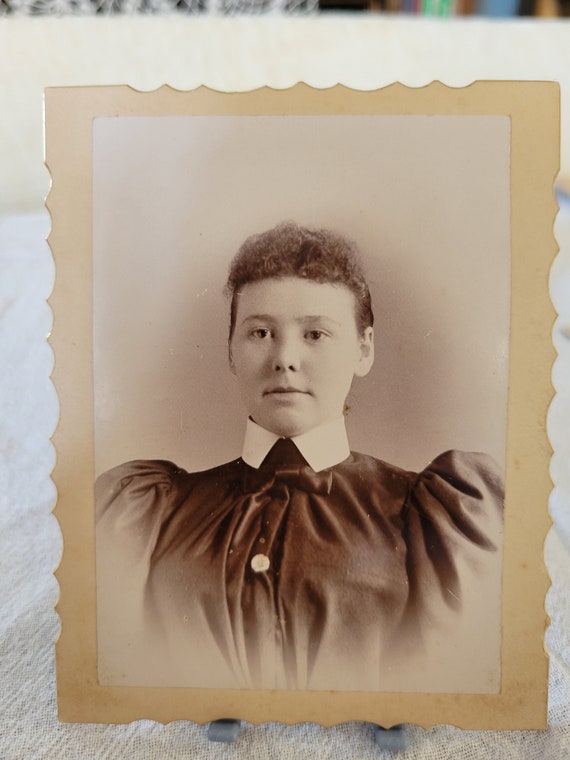The image depicts an old, sepia-toned photograph of a young woman from the late 19th or early 20th century. She is wearing a dark-colored dress with a prominent white collar and a single white button at the chest. The dress features poofy shoulders that rise above her clavicle, and her hair is short, curly, and dark, with a slightly poofy front. The woman appears stoic, looking straight ahead. The photograph is mounted in an off-white, brownish paper frame with wavy, pointed patterns along the edges, which do not extend to the corners. The framed picture is placed on a stand on a white surface, with the top part of the image showing blurry, colorful objects in the background.